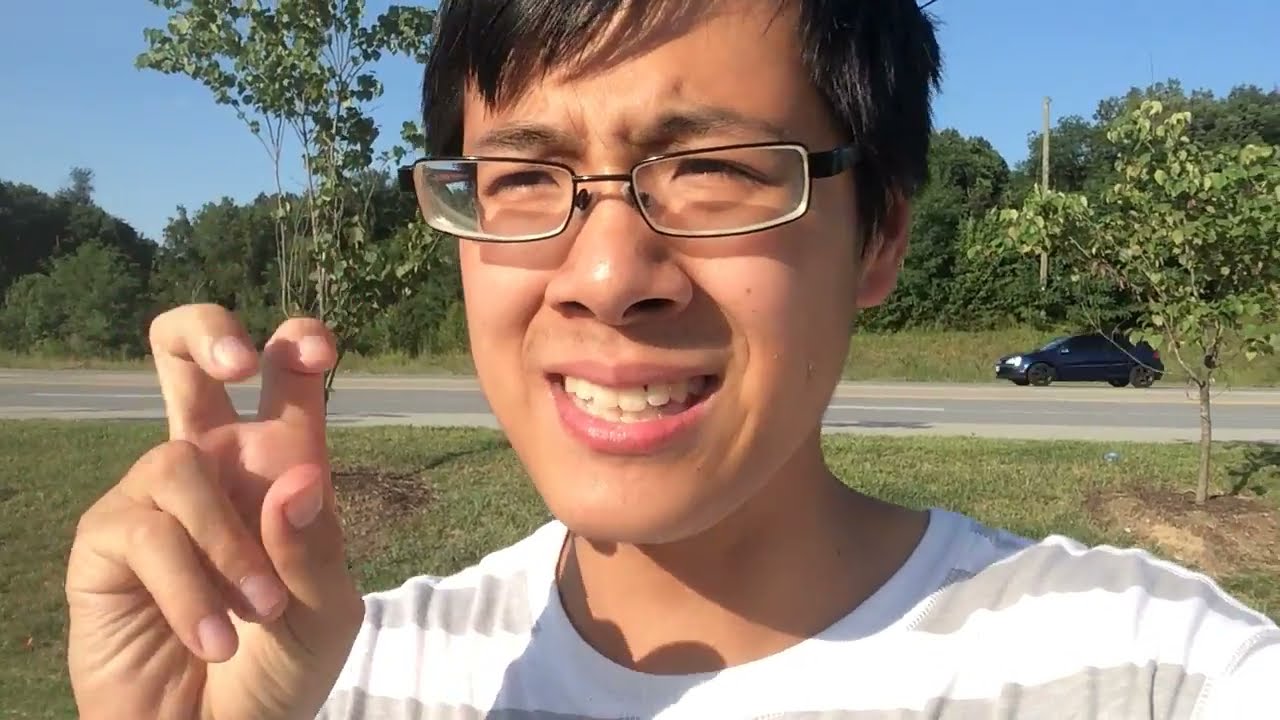In this vibrant photograph, a young Asian male, likely in his late teens or early 20s, stands prominently in the foreground. He sports short black hair and wears rectangular black-framed glasses. His outfit consists of a white shirt adorned with gray stripes. The man exudes joy with a beaming smile that reveals his teeth. He is positioned in a well-maintained grassy area and looks off slightly to the side, adding a candid feel to the image.

Behind him, there is a light-colored asphalt road, free of any vehicles or objects, which divides two patches of mowed grass. Further back, a dense tree line of lush, green foliage stands tall against a clear, cloudless blue sky. The background also features some barely distinguishable object, potentially a rake, almost concealed by the subject. This meticulously composed scene combines elements of nature and tranquility, spotlighting the subject's cheerful demeanor.